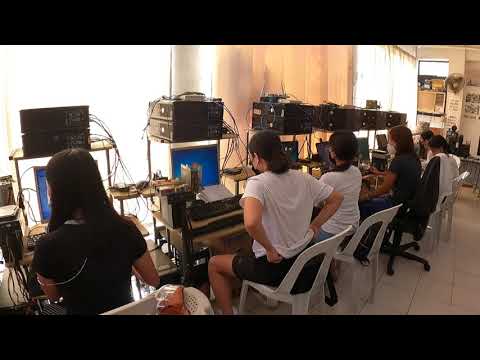The image depicts an indoor classroom-like scene with a group of students, totaling around five to six, seated at desks with computers. They are seated mostly on white plastic chairs, though one is on a black rolling chair. The students, who appear to be predominantly female, have their backs to the camera and are focused on their computer screens, which show minimal activity, likely just the home screen. Each desk has two black computer towers on top. The students are dressed in a mix of white T-shirts and black shorts, with one wearing a black shirt. They all have dark hair and are wearing masks, suggesting the photo was taken during the COVID-19 pandemic. The room is dimly lit due to large windows covered by white curtains, allowing only scant sunlight to filter through. On the right side of the image, there is a bulletin board or picture on the wall, contributing to the minimal décor of the room.